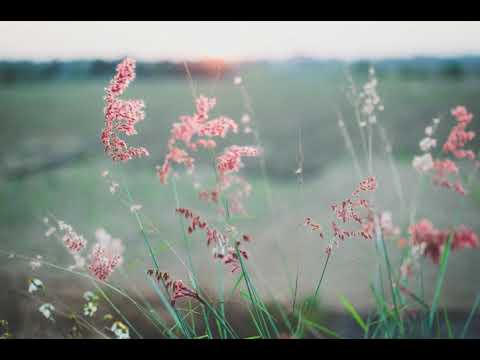A horizontal, nearly square photograph features a striking display of flowers in the foreground against a softly blurred background. There are thin, light green blades of grass with numerous delicate pink flowers clustered along their stems. Some white flowers are also visible, though they appear blurrier than the prominently focused pink ones. The scene in the background is a dreamy, out-of-focus landscape resembling a green pasture or field; the slightly discernible elements suggest patches of varying colors and a line of silhouetted trees meeting the horizon. Above this, the sky transitions into a gentle white, with faint hints of blue hills or mountains. The image is framed by black borders at the top and bottom, enhancing its elongated rectangle appearance.